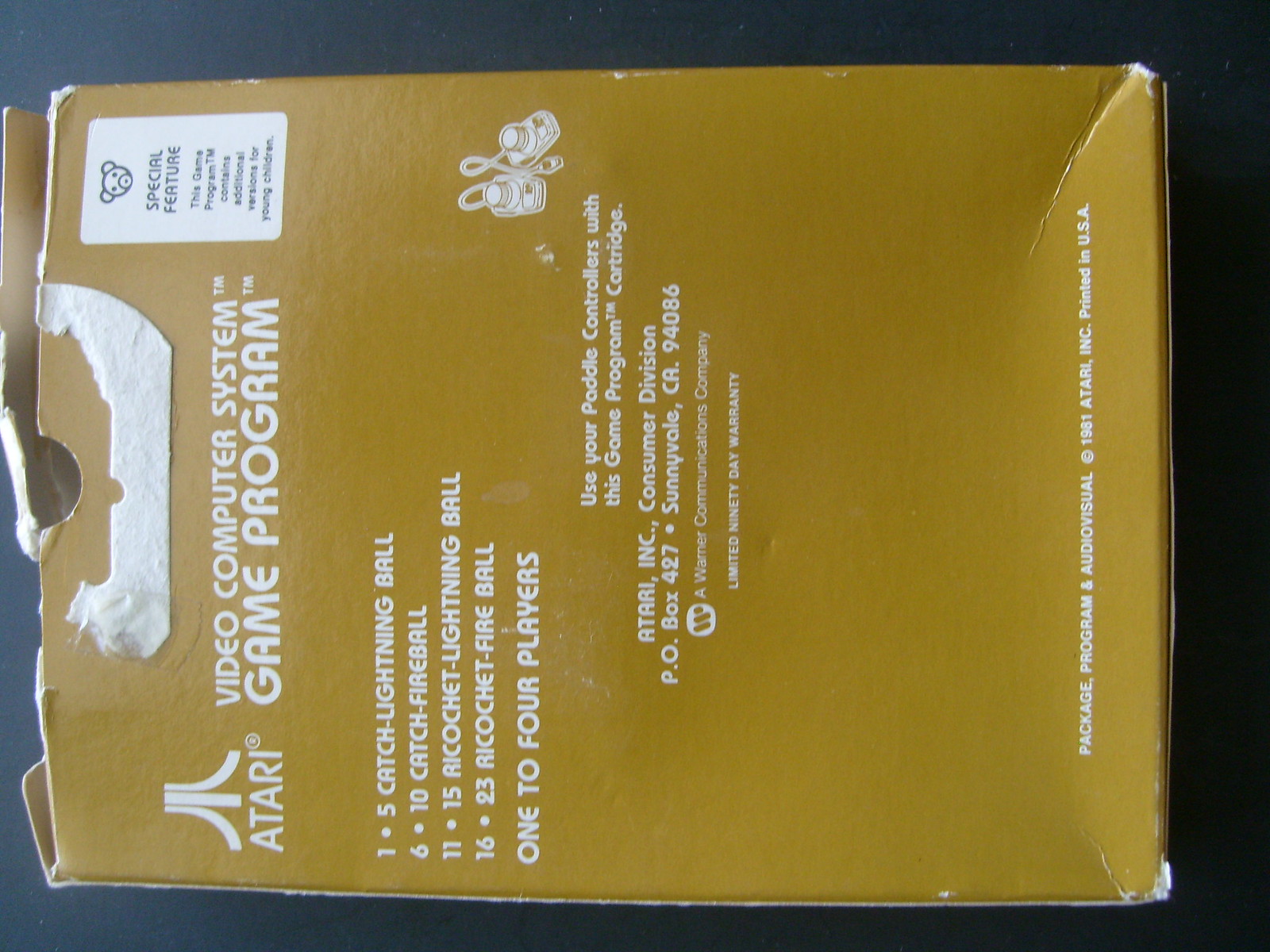The image depicts the back of an Atari video game package, laid on its side, with the front turned to the left. The packaging is a mustard gold color with white text. At the top left, the text reads "Video Computer System Game Program," accompanied by the Atari logo, which features three lines: one long central line flanked by two curved lines. There’s a small white square with a picture of a bear’s head and black text that says "Special Feature," indicating that the game contains additional versions for young children. The box appears slightly creased and wrinkled, and remnants of ripped plastic and cardboard at the top suggest it has been opened. White text on the right side lists game modes, including "1-5 Catch Lightning Ball, 6-10 Catch Fireball, 11-15 Ricochet Lightning Ball, 16-23 Ricochet Fireball," and specifies that the game accommodates "1 to 4 players." The backdrop behind the box is blue, and the image also shows controllers and mentions a Warner Brothers logo.